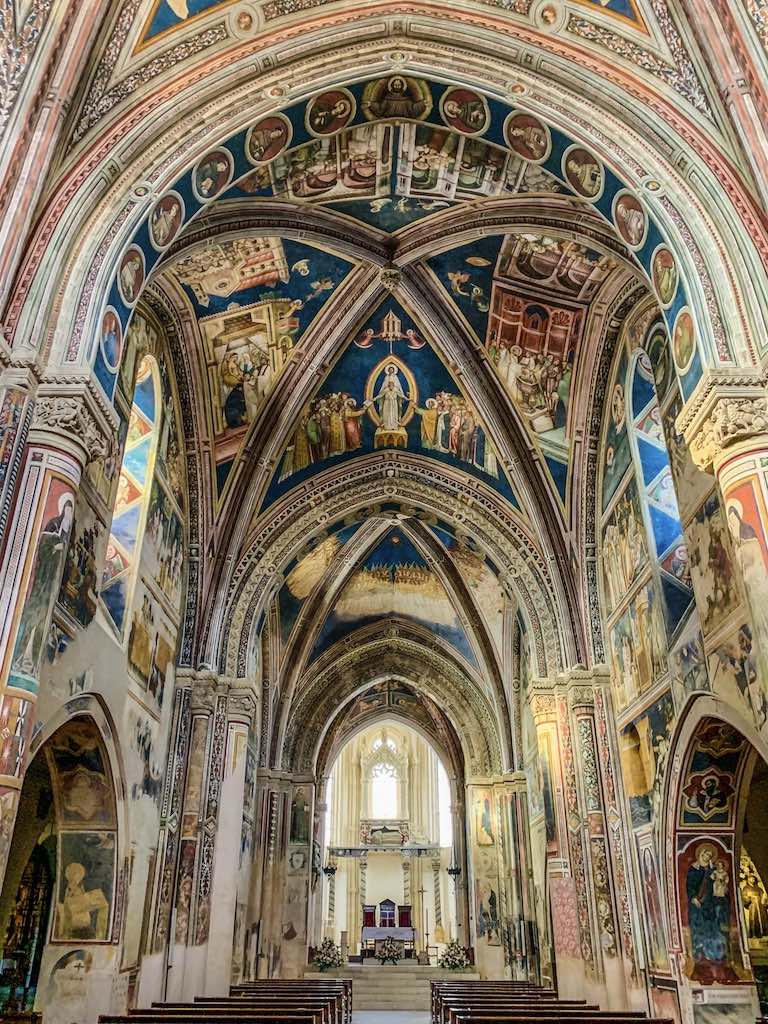This image captures the extraordinarily ornate interior of a medieval Gothic cathedral, characterized by its towering, dome-like ceilings adorned with highly detailed religious murals in dark blue, red, purple, and green hues. The cathedral's ceiling features a star-like pattern of arches that converge with circular portraits of religious figures, including depictions of Jesus, his disciples, Apostles, and angels. Tall arched walls are painted with vivid scenes of religious significance. The space is flanked by dark brown pews arranged in rows on both the left and right, leading towards the altar. At the front, under the soft light filtering through high-placed windows, stands a white altar table accompanied by three high-backed chairs for the priests. There are hints of floral decorations as well, contributing to the sacred ambiance of this possibly ancient and historically significant cathedral.